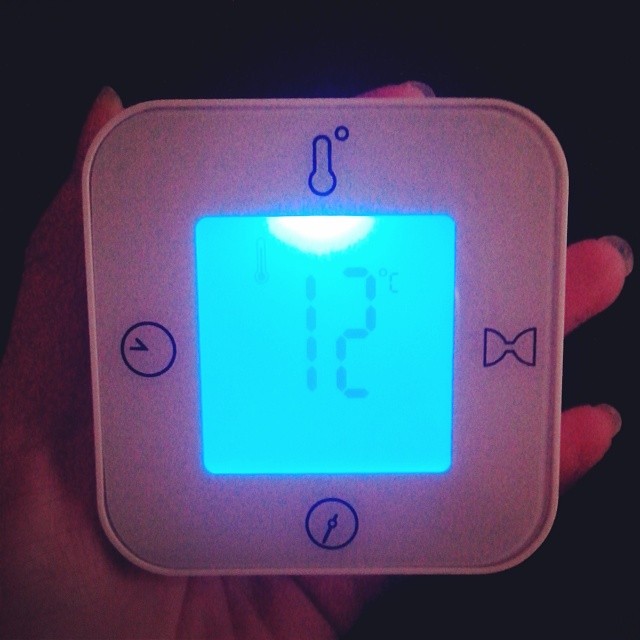This compact, handheld thermostat, crafted from white plastic, features a digital display with a vivid blue background. The current temperature reading is prominently shown as 12 degrees Celsius. In addition to its primary function as a thermometer, this multi-functional device includes several dedicated buttons, each marked with dark blue symbols, for various other features. One button allows you to set a clock, another operates an egg timer, and a third presumably controls a barometer, identified by a circle with a central pointer at the bottom of the display. This versatile tool provides not only temperature but also time and barometric pressure readings, enhancing its utility.